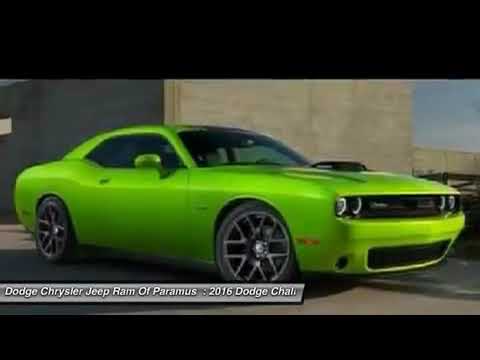This image showcases a vibrant neon lime green 2016 Dodge Challenger, positioned prominently in an outdoor setting. The car’s sleek, brand-new appearance is accentuated by its fancy rims with wider spokes, closed roof, and a small orange taillight. Captured from the right-hand side, the Challenger’s double headlights and partial front view add to its sporty allure. The car is parked on a brown surface in front of a light brown building, with a hint of blue sky visible in the top right corner. Surrounding the photo are two horizontal black strips, one at the top and a narrower one at the bottom. At the bottom left corner of the image appears edited text in white against a gray strip: "Dodge Chrysler Jeep Ram of Paramus: 2016 Dodge Challenger." The detailed and polished presentation highlights the car’s status and design excellence.